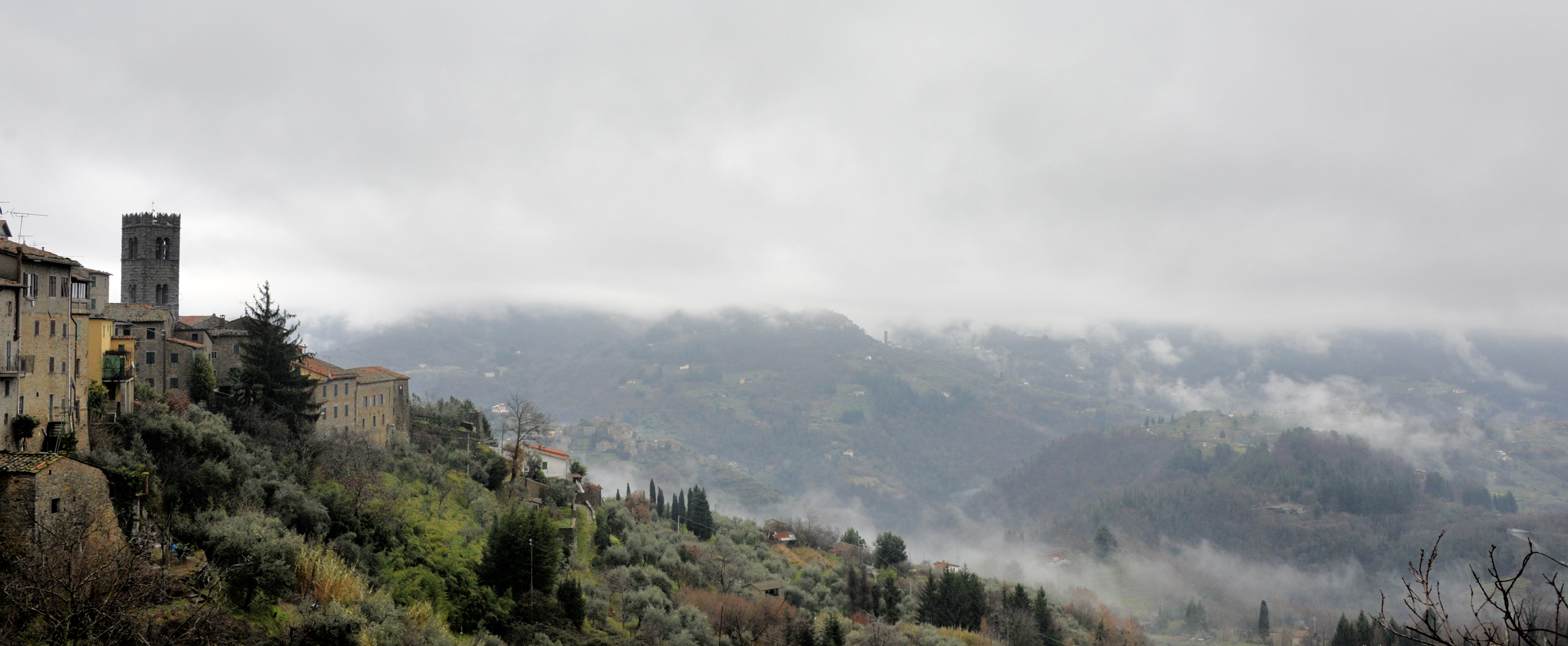A captivating photograph captures a misty hillside that evokes the rustic charm of Southern Europe, possibly Spain, Italy, or France. Dominating the top half of the image, a misty white sky blankets the landscape, lending an ethereal quality to the scene. The hillside itself slopes diagonally from the center left to the bottom right, accentuated by thick bands of fog that cling tenaciously to the ground along the right side of the image.

On the left side, perched prominently atop the hill, stands a stately yellowish-tan stone building, likely dating back to the 18th or 19th century. The structure features a dark brown, sloped roof bristling with several TV antennas on its extreme left corner. The building boasts at least four floors, each lined with rows of windows, adding to its historic allure. Adjacent to its right side, the structure transitions into a gray, square tower reminiscent of an old bell tower, now seemingly repurposed.

As the hill descends, a tapestry of untamed vegetation emerges, with wild weeds, sprawling bushes, and clusters of smaller trees dotting the landscape. Near the center of the image, about halfway down the slope, a quaint white building with a slanted red roof becomes visible, strategically positioned to facilitate optimal water runoff.

Towards the far right corner, an abandoned valley ensconced by dense woods comes into view, shrouded in swirling white fog that further obscures the details of what lies beneath. This abandoned area, covered in a heavy fog, adds a layer of mystery and enigma to this tranquil, dreamlike rural scene.